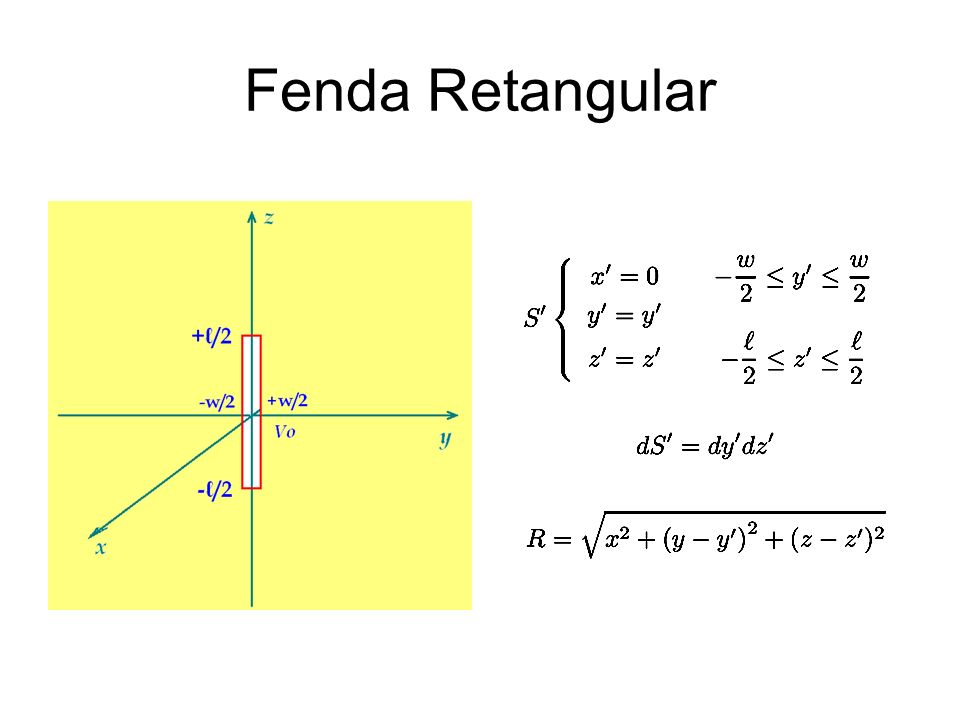The image, labeled as "Fenda Rectangular" at the top in black text, appears to be a detailed slide explaining a complex mathematical concept. The left portion of the image features a prominent yellow square that includes a 3D coordinate system with the Y axis represented by a horizontal green line pointing to the right, the Z axis depicted as a vertical green line pointing upwards, and an X axis represented by another green line inclined downwards to the left from the vertex. Inside this yellow square, there is a small white rectangle annotated with values and axes designations. On the right side of the image, against a white background, there is an array of mathematical equations and formulas written in black text. In the middle section of this white background, there are equations such as "-W/2" on the left and "W/2" on the right. At the bottom, an intricate polynomial is outlined, showcasing "R = √(X² + (Y - Y')² + (Z - Z')²)," which requires further solving. Above this, additional equations like "DS = DYDZ" and "S[X] = 0XYZY" further elaborate the mathematical topic being addressed.